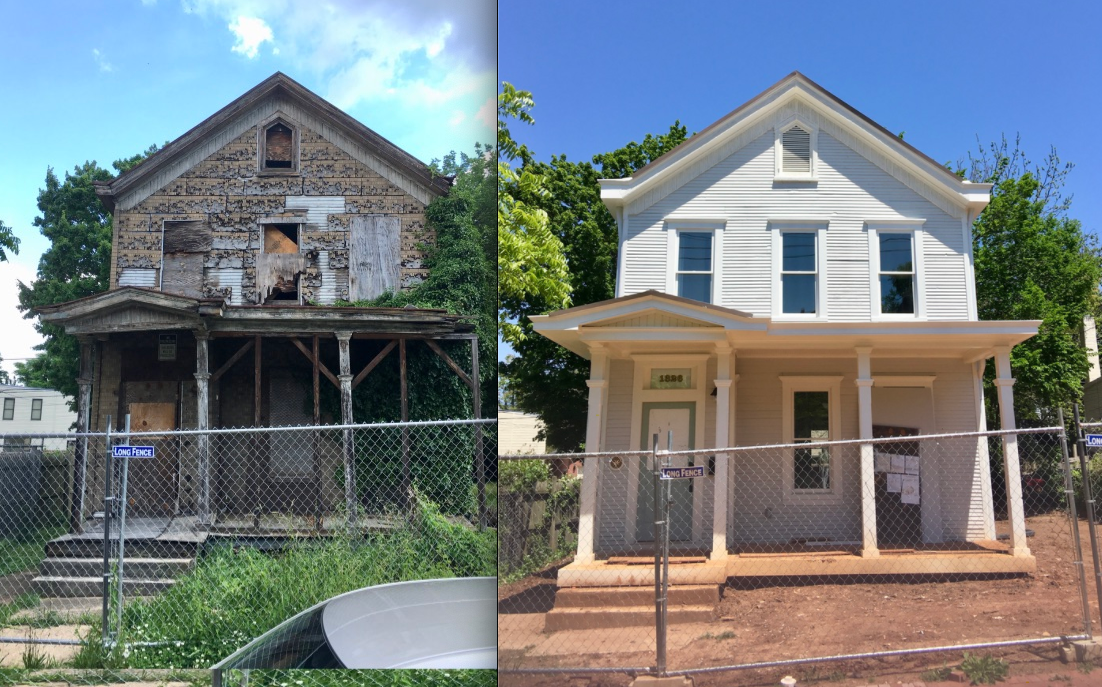The image features two side-by-side photographs of the same house, capturing its dramatic transformation from a dilapidated state to a newly renovated condition. In the left photo, the house appears neglected and run-down with peeling paint and missing trim, giving it a dark and shabby appearance. The exterior is marked by weather-worn columns on the porch, overgrown weeds in the lawn, and an old silver metal fence that's in poor condition. The front door is boarded up, adding to the overall sense of abandonment. 

In contrast, the right photo showcases a stunning renovation. The house now boasts fresh, white trim, a completely repainted exterior, and robust-looking new columns. The formerly weed-filled lawn has been cleared out, likely in preparation for new grass. The metal fence remains but has been restored to complement the house's refreshed aesthetic. The blue sky and green trees in the background are unchanged, further emphasizing the stark transformation of the house itself from its former neglected state to a beautifully renovated home.